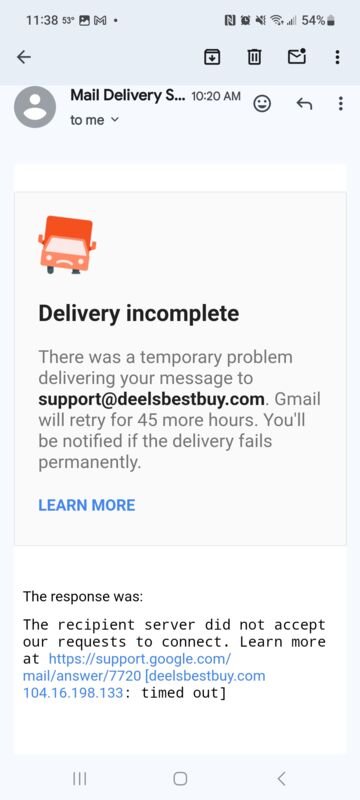The image depicts a cellphone screen displaying an open email message in the user's mailbox. In the top left corner, the number 1138 is visible. The top right corner showcases various status icons, including indicators for cellular connection, wireless connection, and a battery icon showing 54% charge. Directly below these icons, there is a left-pointing arrow followed by additional icons for download (an arrow pointing downward), delete (a garbage can), and an envelope symbol.

On the left side of the email interface, there's a circular icon featuring a profile picture of a person. The email header reads "Mail Delivery S... to me 10:20 AM," accompanied by a smiley face emoji. The main content of the email includes an image of an orange truck with a frowning face, which appears to have a flat tire. In large black text, the email announces "Delivery incomplete." The detailed message states: "There was a temporary problem delivering your message to support@dealsbestbuy.com. Gmail will retry for 45 more hours. You'll be notified if the delivery fails permanently."

Beneath this text, in bold blue uppercase letters, is a link labeled "LEARN MORE." Following this, within a white rectangle, the email further explains: "The response was the recipient server did not accept our request to connect. Learn more at [Google support web address]." Finally, it ends with the term "timed out."